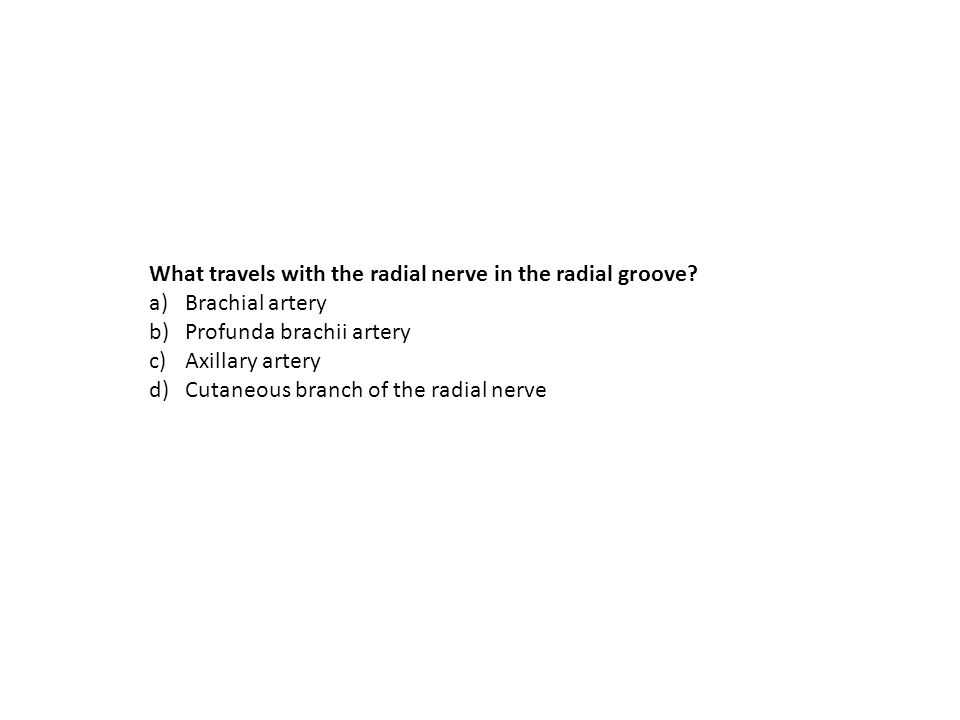The image features a white background with a prominently bold black question at the top left, asking "What travels with the radial nerve in the radial groove?" Following the question are four options labeled in dark gray letters: A) brachial artery, B) profunda brachii artery, C) axillary artery, and D) cutaneous branch of the radial nerve. The text is horizontally aligned and crafted in small, regular print.